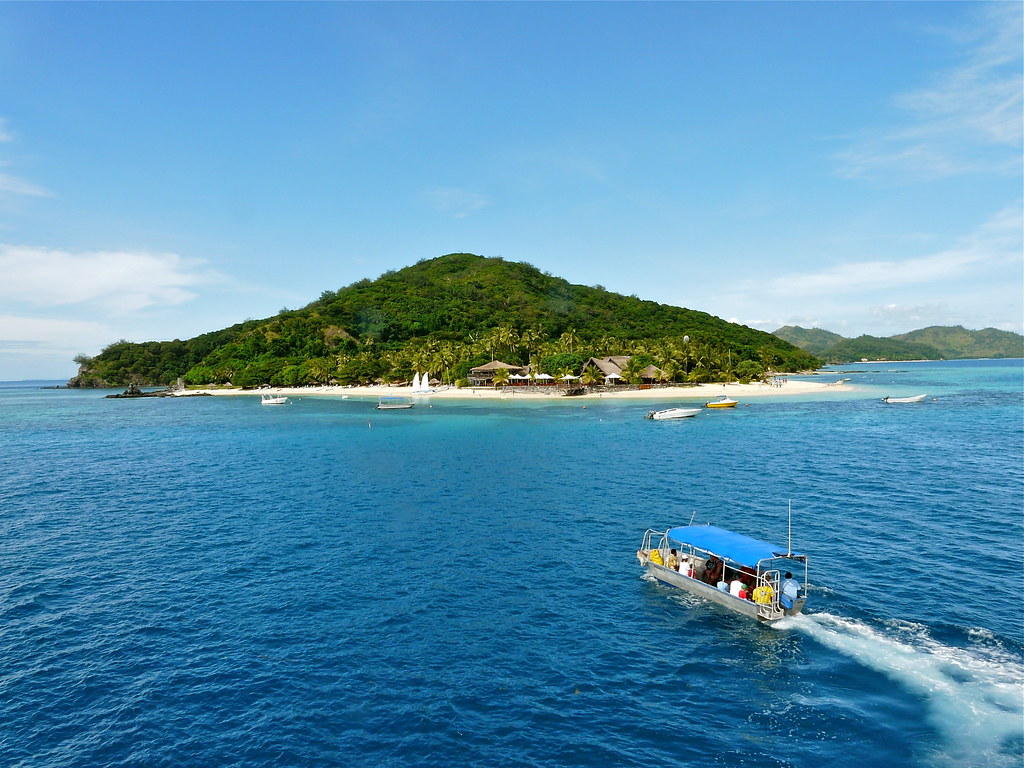This captivating photograph captures a picturesque scene of a serene, expansive body of water. Dominating the foreground is a covered motorboat, reminiscent of glass-bottom boats, teeming with passengers enjoying a leisurely ride. Scattered across the water, numerous small metal boats—likely used for fishing—create a bustling yet tranquil atmosphere. Towards the left of the composition, a graceful sailboat is seen gliding effortlessly, adding a touch of elegance to the scene.

In the middle distance, an inviting island emerges, lush with vibrant green foliage. The island appears spacious enough to accommodate a few tiki huts, accompanied by colorful umbrellas and chairs that suggest a perfect spot for relaxation and social gatherings. Beyond this primary island, several smaller islets dot the horizon, their green vegetation hinting at untouched natural beauty, but lacking the expanse for development. This idyllic setting showcases a harmonious blend of human activity and pristine nature, inviting viewers into a serene aquatic paradise.